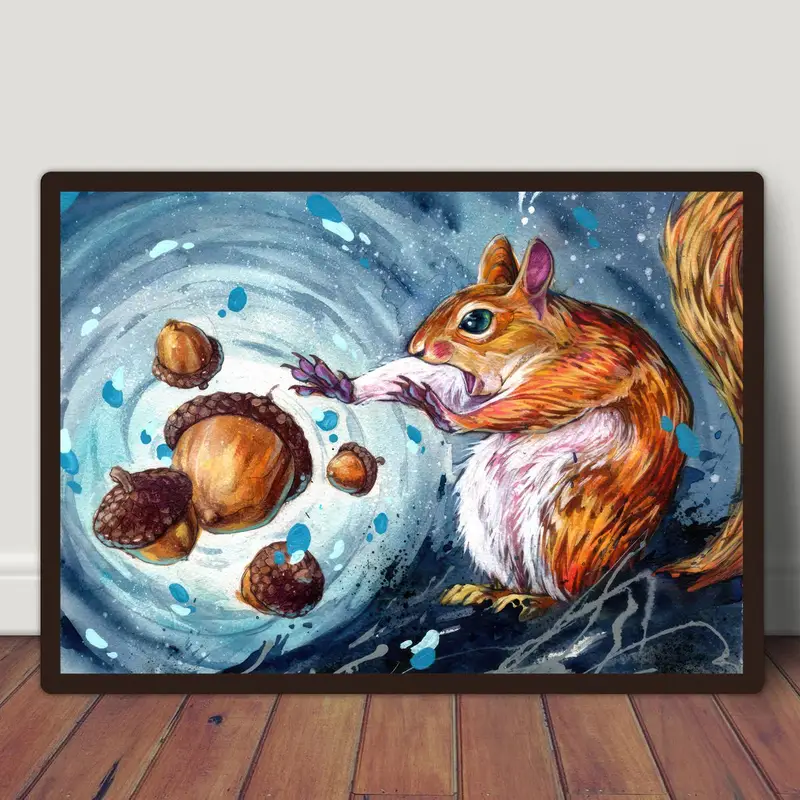The artwork depicts a humorous scene featuring a brown squirrel with a surprised, wide-eyed expression, reaching its paws out toward a swirling vortex of acorns. The squirrel, characterized by its brown fur, white chest, and green eyes, stands out vividly against a predominantly blue and white, wind-swirled background, which gives the impression of motion and chaos. The acorns, numbering about five or six, are caught in this whirl of air, adding to the frantic energy of the scene. The piece is framed in black and positioned against a light gray or white wall, resting on a medium-brown, wide-planked wooden floor. The overall effect conveys the squirrel's astonishment and the swirling energy of the acorn-laden vortex.